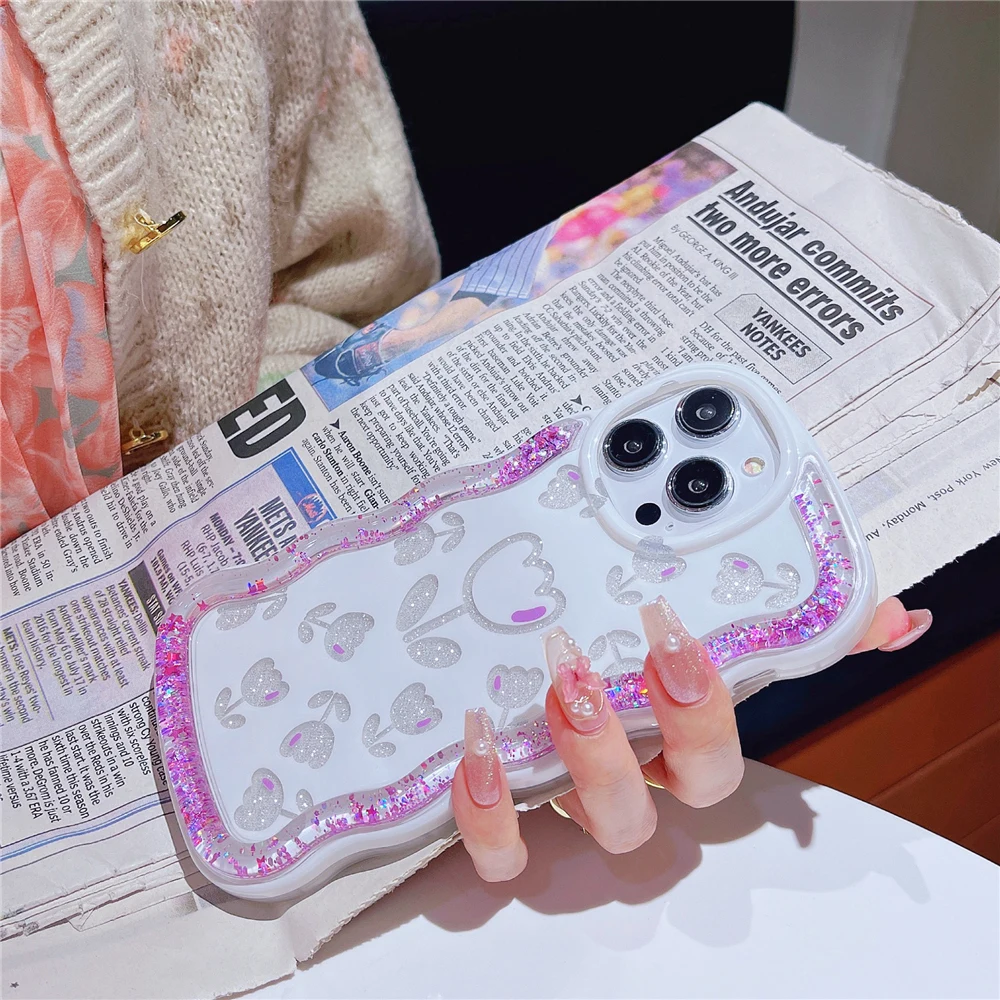A detailed image shows a woman holding a white iPhone with an ornate, glittery case in one hand and a folded newspaper in the other. The phone case features a raised plastic design with silver tulip-like flowers and purple glitter around the edges, alongside three visible camera lenses. The woman's fingernails are long and meticulously manicured, painted with a clear pink polish adorned with pearls, glitter, and pink butterfly stickers. Her fingers, visible up to the knuckles, are thin and delicate. She is dressed in a light-colored, possibly vintage, knitted sweater with gold buttons. Beneath the sweater, she wears a peach-colored floral shirt with pleats. There is also a glimpse of her white skirt or pants. The newspaper she holds features articles about the New York Yankees. In the bottom right of the image, part of a wooden surface is visible. The woman is seated on a brown bench.